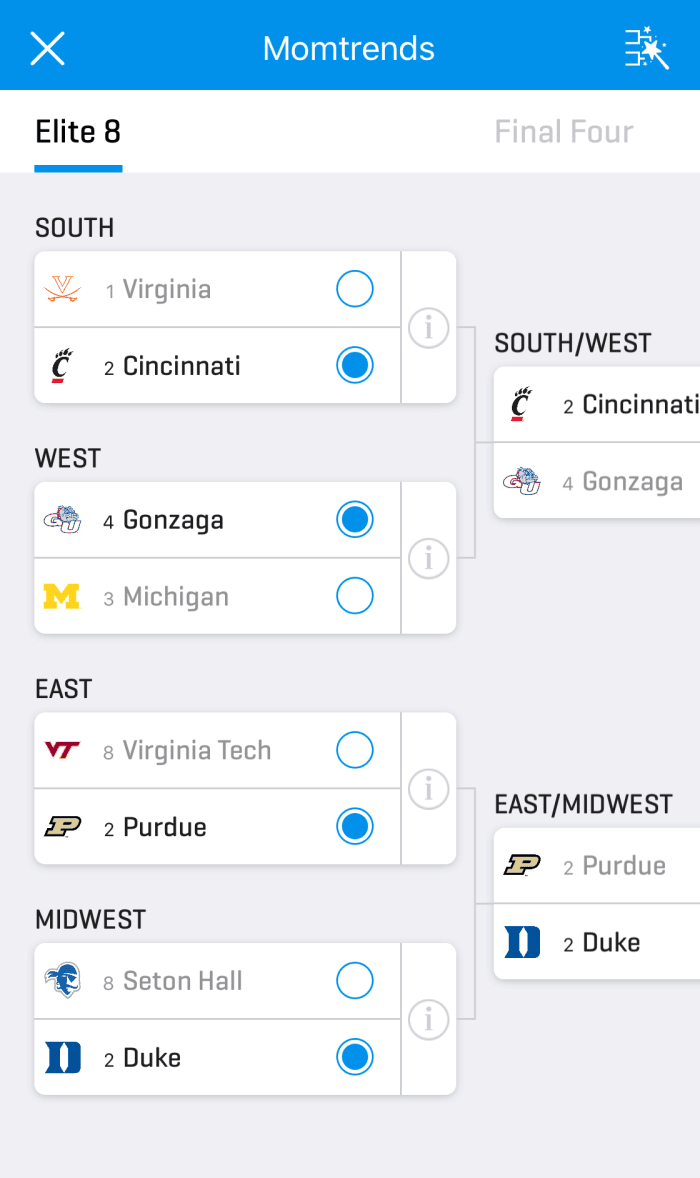**Caption:**

A detailed playoff bracket for a college football tournament, prominently labeled "Mom Trends" at the top. The bracket highlights the Elite 8 teams, which include Virginia, Cincinnati, Gonzaga, Michigan, Virginia Tech, Purdue, Seton Hall, and Duke. Advancing from the Elite 8, Cincinnati and Gonzaga faced each other, with Cincinnati emerging victorious. In parallel, Purdue and Duke clashed, with Duke securing the win. The Final 4 teams were thus Cincinnati, Gonzaga, Purdue, and Duke. Ultimately, Cincinnati and Duke advanced to the championship game.